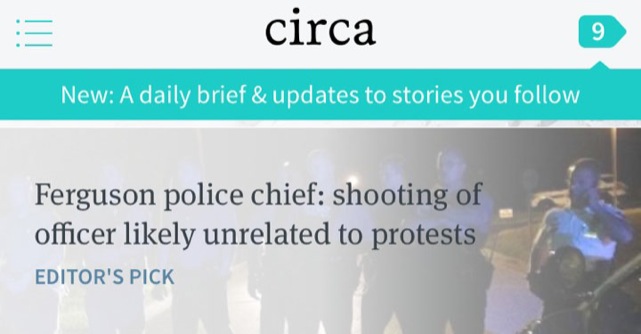This image showcases a webpage from a news site named "circa." At the top of the page, there's a blue button alongside black text that reads "circa," both positioned on a blue background, which also features the number "9." Adjacent to this is a label marked "new."

The webpage highlights a section titled "A daily brief and updates to stories you follow." Below this, an article headline reads, "Ferguson Police Chief: Shooting of officer likely unrelated to protests," with the label "Editor's Pick" in blue text.

The background image depicts a nighttime scene with several police officers. The dark sky suggests it is night, and there are police cars visible in the distance, their lights gleaming. The officers, approximately six or seven in number, are wearing what appear to be white uniforms and are standing in a circular formation. Some of them seem to be holding helmets. This image serves as the backdrop, while most of the page foreground is dominated by the text and various labels of the website.